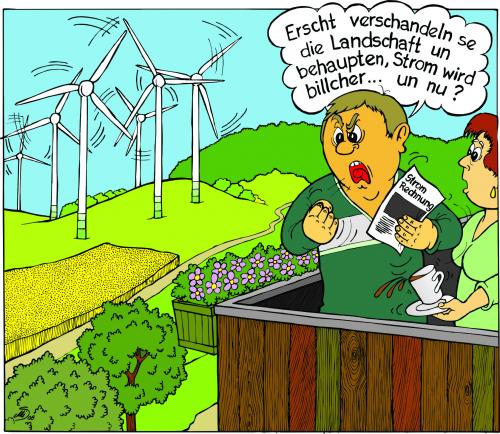In this detailed cartoon drawing, the scene is set in a vibrant garden with a light and bright green grassy landscape. On the bottom left, there are two green bushes adjacent to a planter bursting with pink flowers. The left side of the image is dominated by a picturesque landscape of green hills dotted with white windmills spinning and seemingly forming a wind farm.

On the right side, a couple stands on a balcony made of horizontal or vertical wooden planks, which also features a flower box. The man, appearing very angry, is wearing a green shirt and has mustard green hair. He clutches a piece of paper labeled "Stromrechnung" (electricity bill). He is shouting something in German, potentially about the cost of electricity. His wife, standing to his right, wears a light green dress and has brown hair. She appears startled and is spilling her white cup of tea or coffee, possibly in response to his outburst. The setting conveys a sense of rural tranquility contrasted with the man's evident frustration.